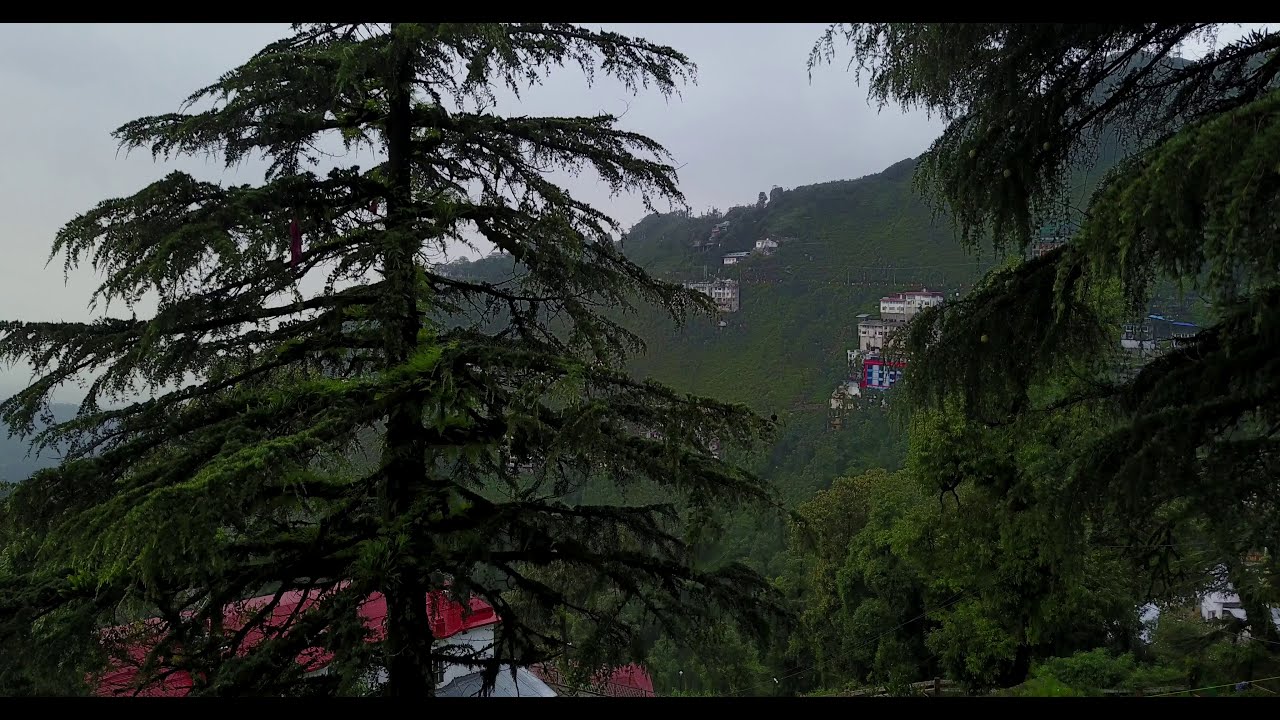The photo captures a lush, green mountain with several houses and building units scattered across its sides. The mountain is heavily vegetated, obscuring any rocky surfaces, and the entire scene is dominated by dense plant life. Prominently featured in the foreground on the left is a large, old tree, seemingly dead but covered in vibrant green moss. Behind this tree, a red-roofed structure can be partially seen. The overall atmosphere of the image is shrouded in gray smog, suggesting a cloudy day with limited visibility of the sky. The houses are positioned throughout the image, appearing in the bottom left, bottom right, center right, and center top areas, illustrating a spread-out, rural settlement clinging to the mountain face. The scene is devoid of text and includes a color palette of grays, whites, greens, browns, reds, and blacks.